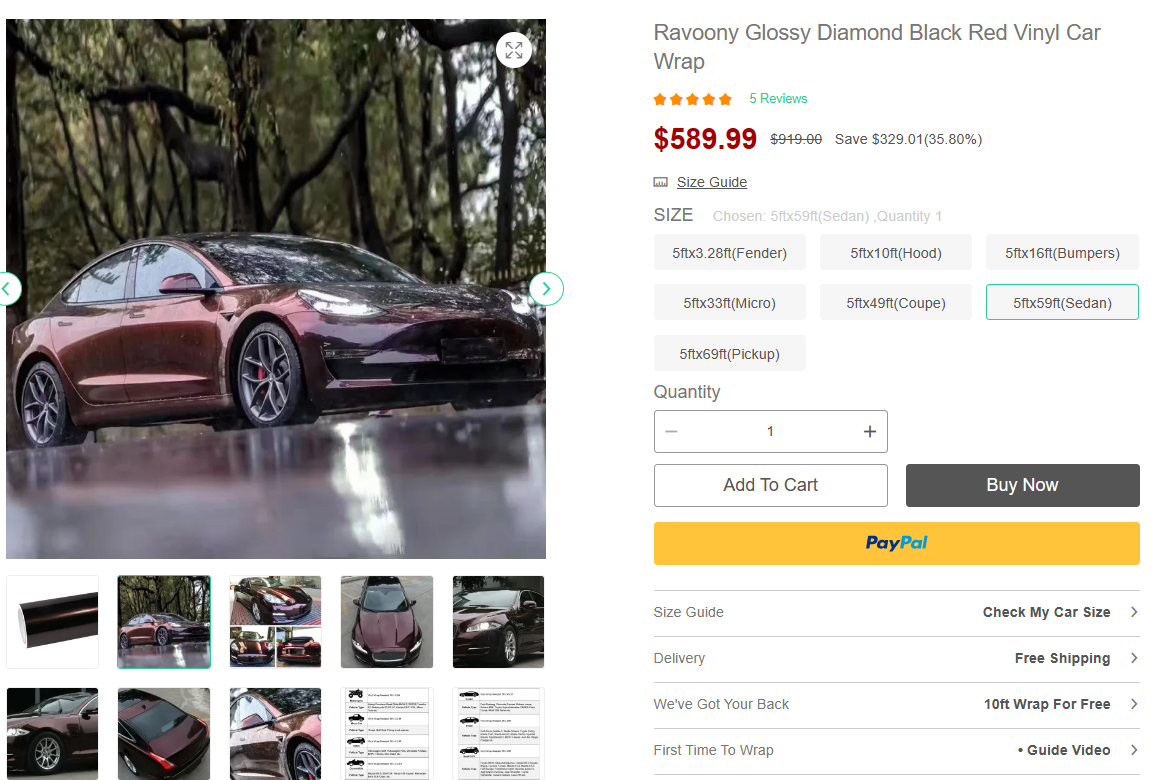A striking image presents a vibrant red car positioned in a serene wooded area, capturing potential buyers' attention. Below the main image, there are several smaller photos showcasing various angles of the vehicle. On the right side of the layout, detailed information is highlighted: "Ravooni Glossy Diamond Black Red Vinyl Car Wrap," priced at $589.99. The size guide specifies dimensions for various sections of the car, including options for fenders, hood, bumpers, micro, coupe, sedan, and pickup, ranging from five feet by three feet to five feet by 69 feet. A user-friendly interface offers quantity adjustment, 'Add to Cart,' 'Buy Now,' and a yellow 'PayPal' button for immediate purchases. Additional features include a size guide checker tool, delivery details, free shipping offers, and an introductory guide video for first-time wrappers. The white background emphasizes the product images and text, ensuring clear and accessible information. Thank you for watching.